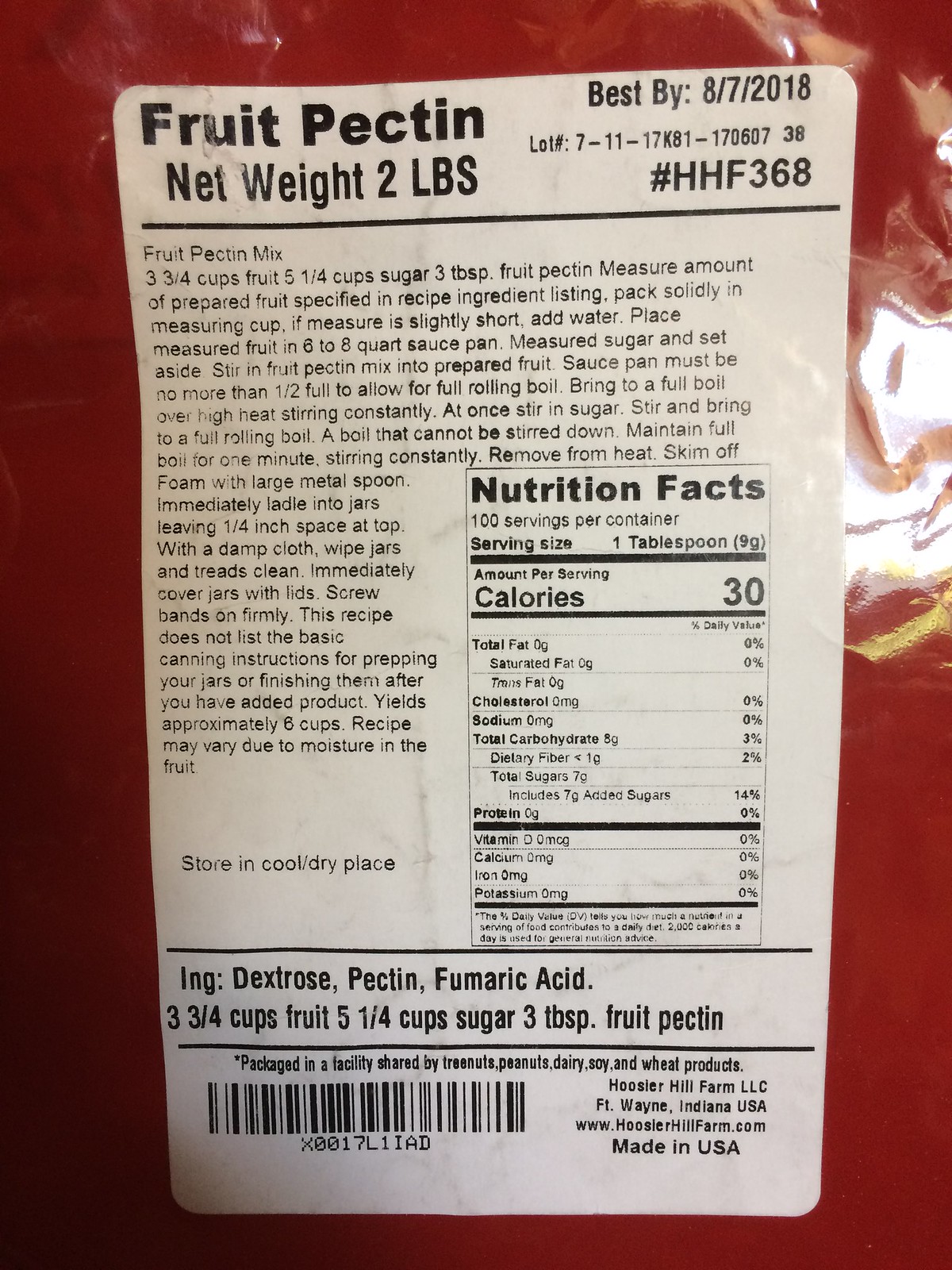The image showcases a detailed label on the packaging of fruit pectin, with the packaging itself being plastic and predominantly red in color. The label is white and contains various bits of crucial information in clear, concise text.

At the very top of the label, it states "Fruit Pectin," followed by "Net Weight 2 pounds" and a "Best By Date of 8-7-2018." A specific lot number is also indicated. Directly beneath this, there is an extensive recipe for making a fruit pectin mix, providing detailed instructions for those who wish to use the product for cooking or baking.

The nutrition facts section reveals that one tablespoon of this fruit pectin contains 30 calories, and the entire container holds approximately 100 servings. 

Further down on the label, the ingredients are listed as dextrose, pectin, and fumaric acid. The recipe specifics include "3-3/4 cups fruit, 5-1/4 cups sugar, and 3 tablespoons fruit pectin." There is also an allergy warning stating that the product was packaged in a facility that processes tree nuts, peanuts, dairy, soy, and wheat.

The label concludes with the manufacturer’s information: "Hoosier Hill Farm, LLC, Fort Wayne, Indiana, United States." Their website, "www.hoosierhillfarm.com," and the indication that the product is "Made in the USA" are also prominently displayed.